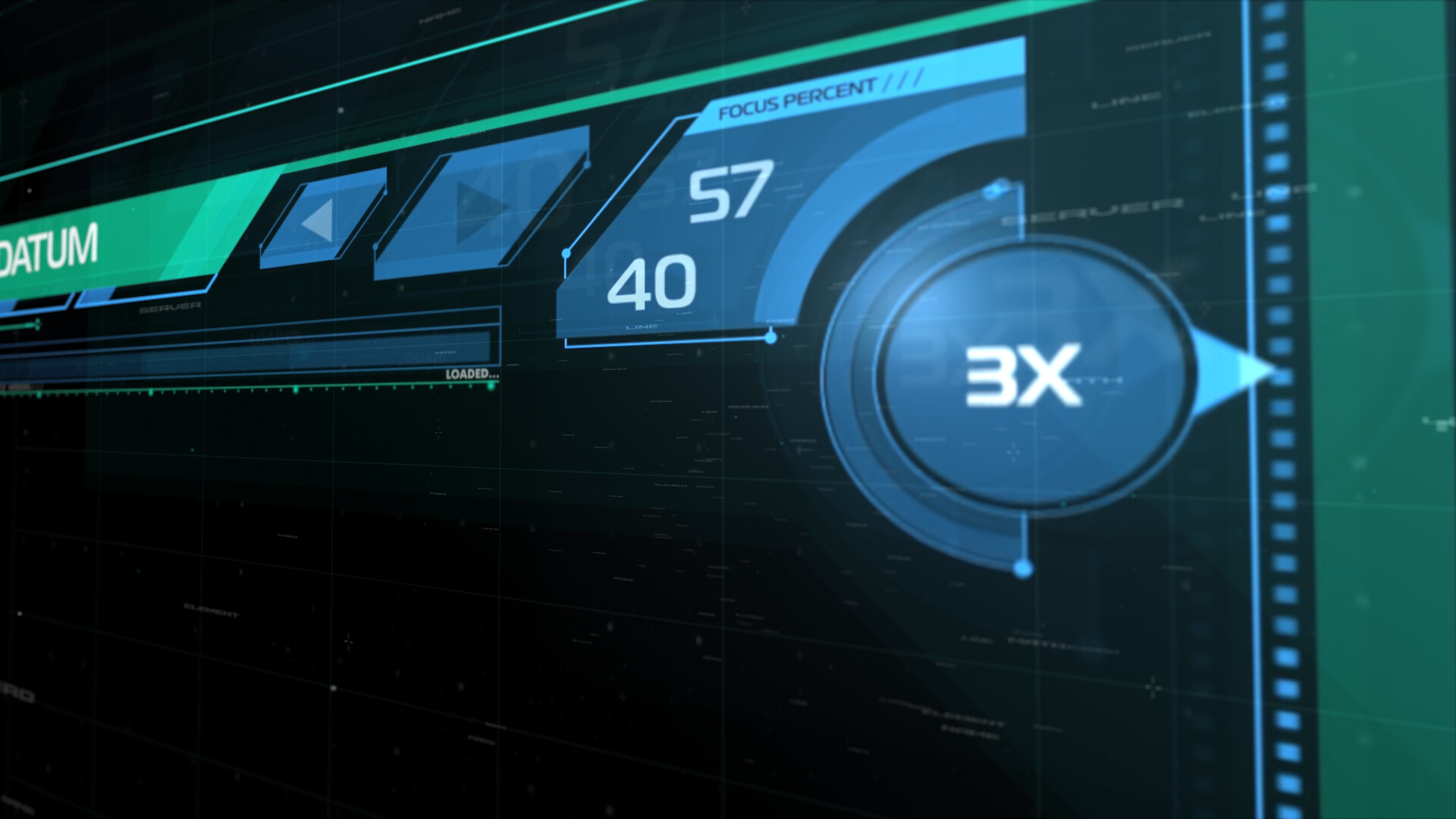This photograph captures a detailed close-up of a digital HUD or user interface on a black screen accentuated with blue, white, and green elements. Dominating the right side is a blue circle framed by a black and blue ring, featuring a right-pointing white arrow labeled "3X." Enclosed within the circle are white numbers. Adjacent to this, a segmented area reads "Focus Percent," displaying the numbers 57 and 40. To the left of this, two arrow buttons are visible: the left-facing arrow is highlighted, while the larger right-facing arrow appears inactive. Below this arrangement, a progressively shrinking bar labeled "Loaded" extends towards the left. Additionally, a green bar in the top left corner contains partially visible white text, cut off to display only "O-A-T-U-M."